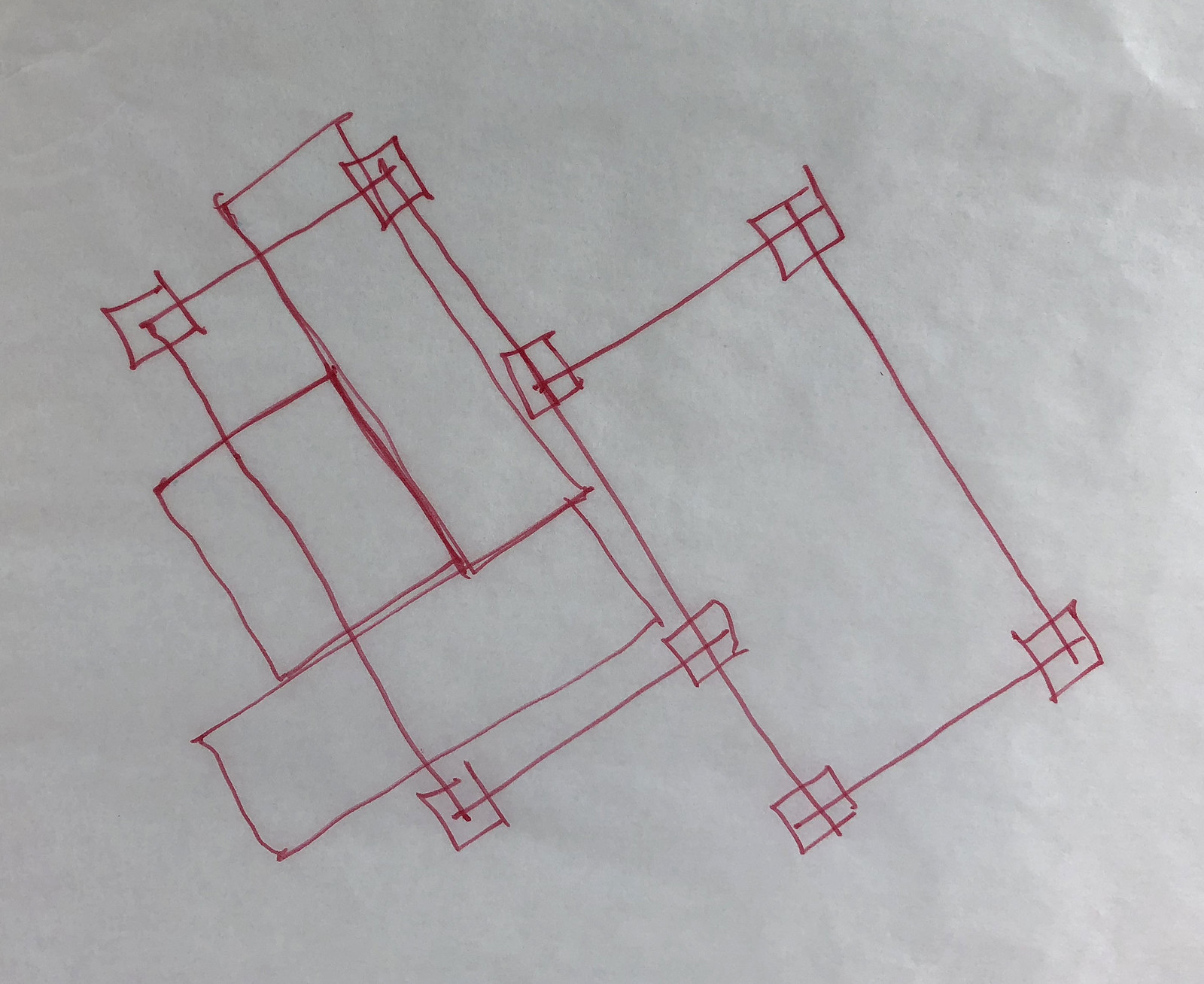This image depicts a hand-drawn red pen sketch of a building blueprint on shiny white paper, resembling greaseproof paper. The drawing shows a building in a crude, diagonal outline. On the right-hand side, there's a rectangular structure marked with small squares at each corner, suggesting potential support columns or corner details. To the left of this building and positioned slightly forward, another long rectangular shape is drawn. Below this shape, perpendicularly aligned, is another rectangle. Overlapping these three rectangles on the left side, there's another structure of similar size and shape to the initial rectangle, also marked with small squares at the corners. The sketch is noticeably untidy, with uneven lines and multiple overlaps, reflecting a rough draft or initial concept phase.